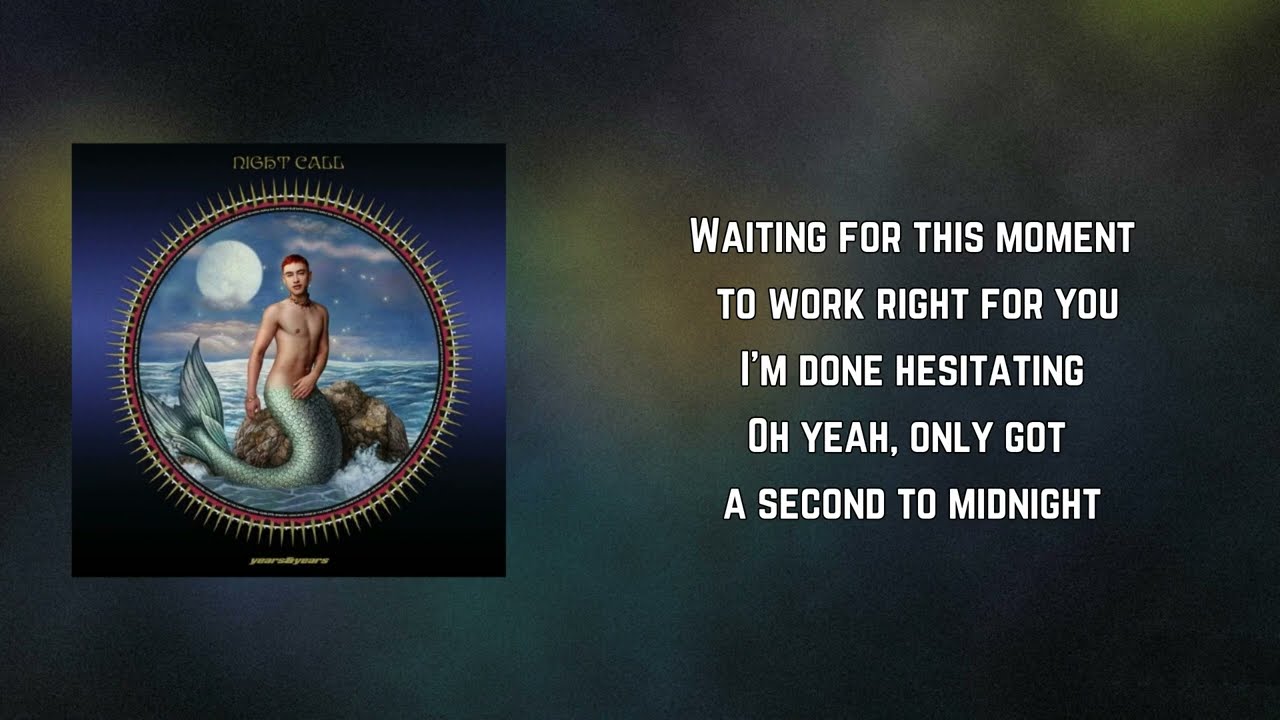The image features an album cover titled "NIGHT CALL," prominently displayed above a striking scene of a man-mermaid, or merman, seated on a brown rock in the middle of a blue ocean. The background transitions from a dark blue at the top to a lighter blue at the center, giving a gradient effect that frames the central figure beautifully. Encircling the merman is a symmetrical circle adorned with gold, almost orange spikes radiating outwards.

The merman, who has cropped red hair and a bare chest, is seen with one hand covering his groin and the other hanging down beneath his hip. His green tail swoops gracefully to the right and then arcs back to the left, with one part of the tail pointing up towards a moon in the background on his upper left side. The sky behind him is adorned with clouds, adding a mystical quality to the scene.

On the right side of the poster, in white uppercase letters, is a compelling text that reads, "WAITING FOR THIS MOMENT TO WORK RIGHT FOR YOU, I'M DONE HESITATING. OH YEAH, ONLY GOT A SECOND TO MIDNIGHT." The overall composition is dark blue at the edges, further highlighting the central elements and the ethereal atmosphere of the album cover.